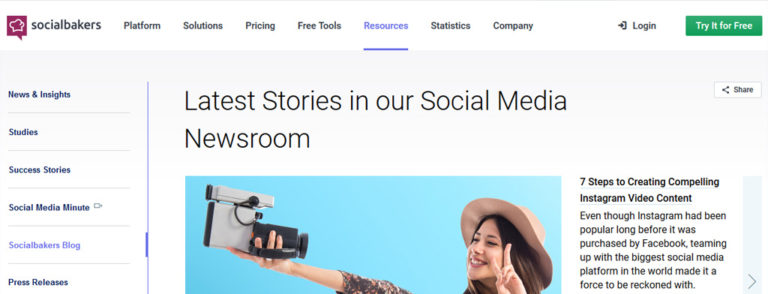In the top left corner of the image, there is a purple text box featuring a baker's hat in the center, labeled "Social Bakers." Below this box is a horizontal menu with options that read from left to right: Platform Solution, Pricing, Free Tools, Resources, Statistics, Company, Login, and Try it for Free. Directly beneath this menu, a gray box offers additional categories: News and Insights, Studies, Success Stories, Social Media Minute, Social Bakers Blog, and Press Releases. To the right, bold black letters announce "Latest Stories in our Social Media Newsroom," accompanied by a share button.

The main image below these text elements has a blue background and showcases a woman wearing a wide-brimmed hat. She is holding an old-fashioned video camera and flashing a peace sign at the camera. The text on the image reads: "Seven Steps to Creating Compelling Instagram Video Content." An accompanying blurb mentions that Instagram, popular long before its acquisition by Facebook, became an influential player in the social media landscape after teaming up with the world’s largest social media platform.